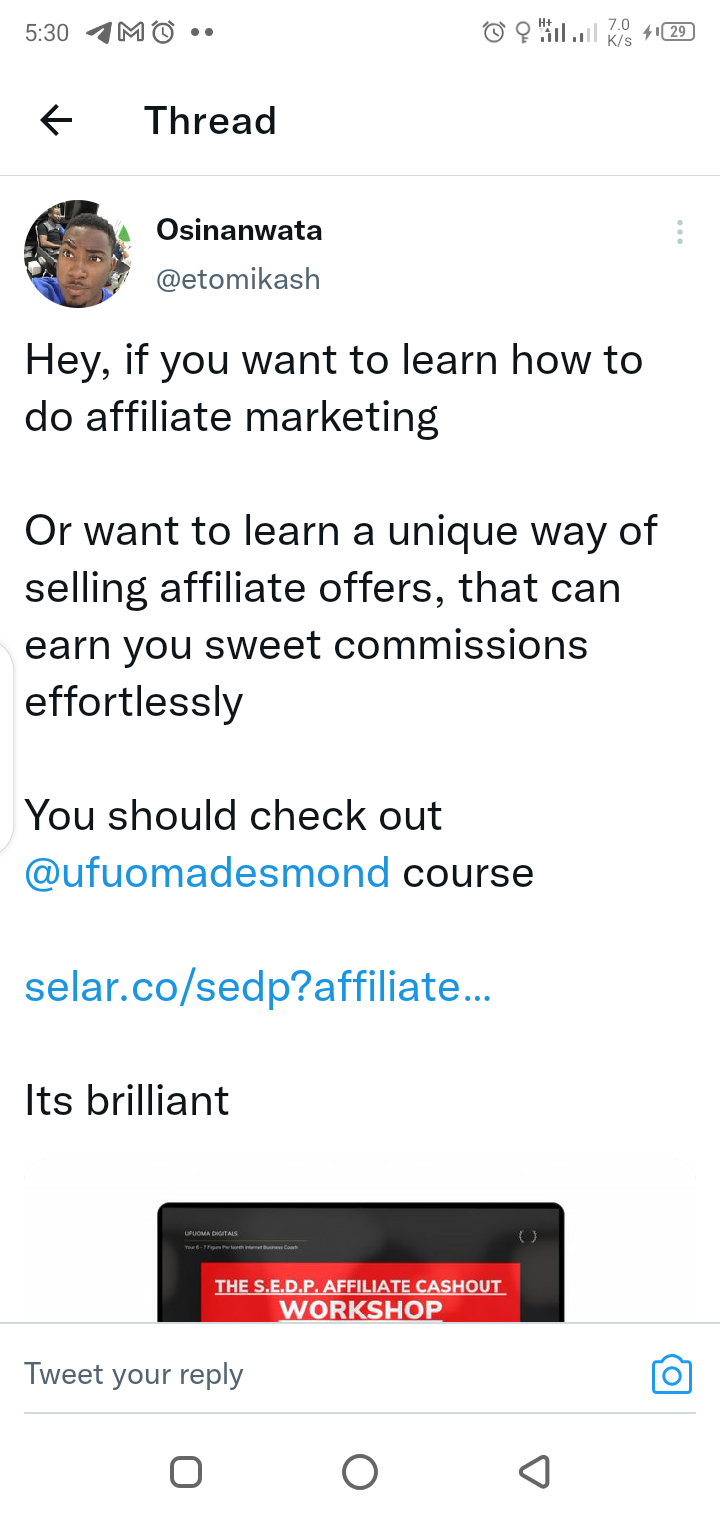The image displays a smartphone screen with several elements arranged in a typical messaging app interface. At the top, the numbers "530" are prominently shown, indicating the time. Directly below is the word "Thread" with an arrow pointing to the left, signifying navigation back to the thread list. The top bar also features a clock icon, a Telegram icon, an alarm clock icon, and a signal strength indicator showing two out of four bars. Unfortunately, the remaining battery life is unclear.

Beneath these icons, the screen shows a section with a profile picture of a Black man wearing a blue shirt. The name "Osinonwara" appears next to the picture, and "Itomikosh" is displayed right below the name. The message from Osinonwara reads: 

"Hey, if you want to learn how to do affiliate marketing, then..." 

The message skips a line and continues:

"I want to learn a unique way of selling affiliate offers that can earn you sweet commissions effortlessly." 

Another gap is left before the concluding suggestion:

"You should check out [Ufuma Desmond's course](Solar.co/sedp/affiliate...)"

Both "Ufuma Desmond's course" and "Solar.co/sedp/affiliate..." are clickable blue hyperlinks, likely leading to further information on the affiliate marketing course.